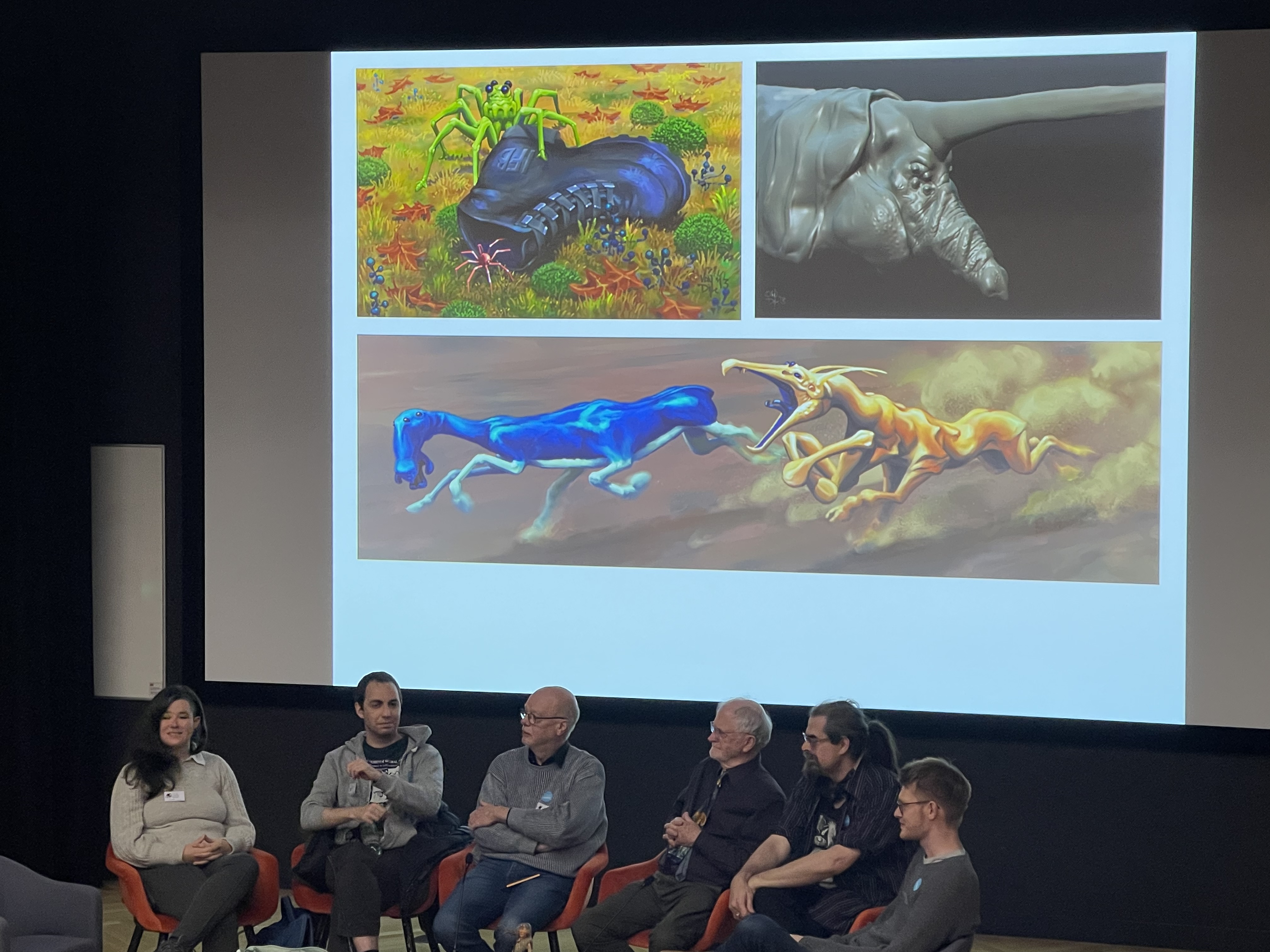In this image, we see a professionally staged conference or panel discussion with six individuals seated on reddish-orange chairs, side by side. Each person appears to be wearing a name tag, indicating their formal role in the event. The panel consists of five males and one female. The two older males, possibly in their 60s or 70s, are indicated to be around 80 years old and one of them is noticeably bald. Among the younger males, one has a ponytail and another one is wearing glasses. The group is a mix of casual and formal attire, with at least one man donning a shirt and tie.

The background features a large projector screen displaying three distinct sub-images of various animals. The top-left image illustrates a vivid and fantastical scene with a green, cartoon-like spider atop a boot in a field, alongside a smaller pink spider. The top-right image shows a grey rhinoceros-like creature with a shell and a lengthy horizontal horn against a grey backdrop. The bottom image portrays two animated, modern-style animals racing in a dusty terrain; one is blue with a long neck and an unusual head, while the other is yellow with a head resembling a pterodactyl.

The ambiance of the photograph suggests a blend of formality with quirky artistic elements, capturing a moment of intellectual exchange amidst an imaginative visual setting.